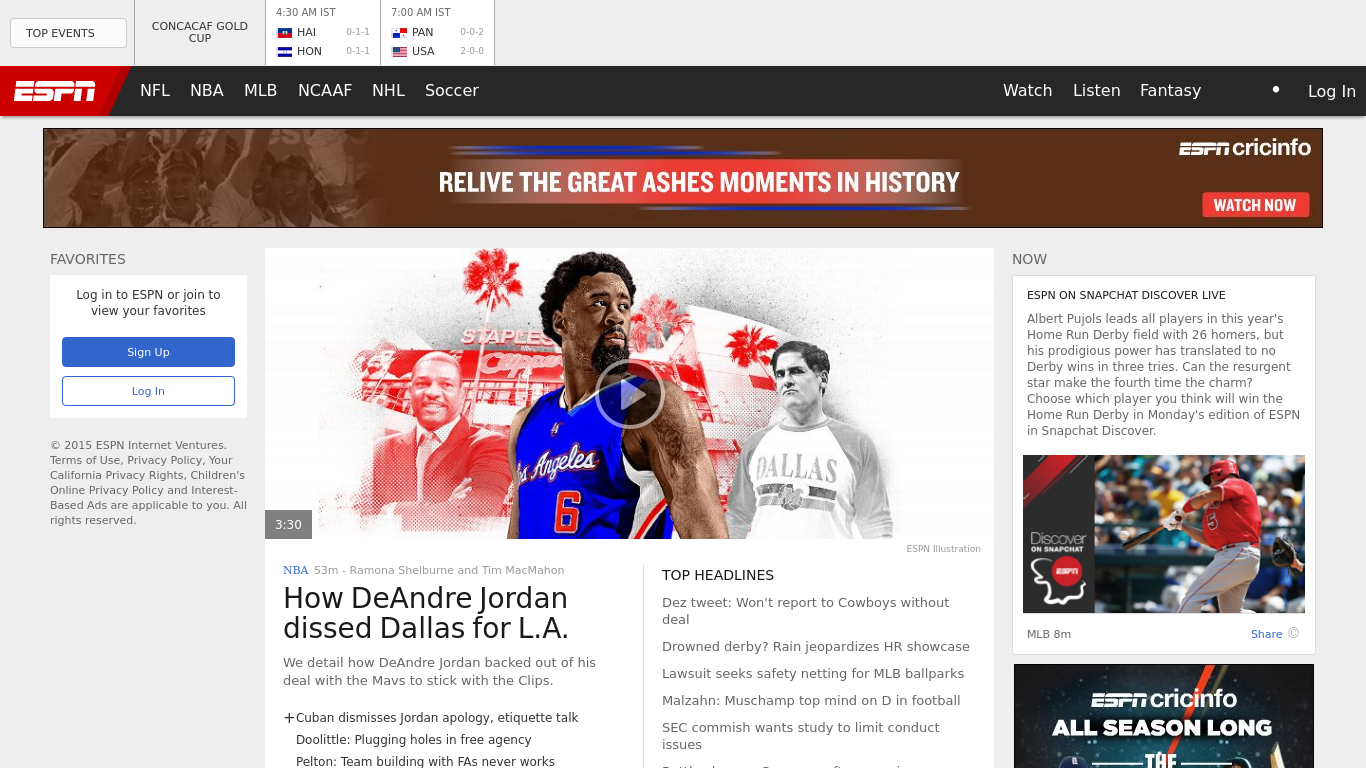Here's a polished and detailed caption for the image based on the provided description:

---

A screenshot from the ESPN website showcases a navigational and content-rich layout. At the top, a gray border frames the site, with "Top Events" listed on the upper left. Adjacent to this, within a white square, are various scores and a reference to the Gold Cup. Just below, a dark horizontal band spans the width of the page, featuring the ESPN logo on a red background towards the left. This band includes white text for key sports categories such as NFL, NBA, MLB, NCAAF, NHL, and Soccer, each separated by the black background.

To the far right of this dark band, options like Watch, Listen, Fantasy, and Login are displayed. Beneath this, a wide brown band continues horizontally. On the right side of this band, the word "ESPN" appears followed by "Cricinfo" while, centrally positioned, there’s a prompt to "Relive the great Ashes moments in history." Below the "Cricinfo" label, a red rectangle with white text invites users to "Watch Now."

The main focus of the screen is a central image beneath the brown band, depicting a Los Angeles basketball player, wearing a royal blue jersey with a red number 6, emblazoned with "Los Angeles" across the front. To the right of this player, a man in a black and white outfit with a Dallas shirt is featured. On the left of the basketball player, an image shows a suited man from the chest up, smiling at the camera with a backdrop suggesting the Staples Center.

Below this composite image are two columns. The prominent headline reads "How DeAndre Jordan dissed Dallas for L.A." followed by a few lines of explanatory text. In the adjacent column, under "Top Headlines," are around five or six news lines. To the left of the main image, a "Favorites" column stands out against a gray background, showcasing a white square with blue rectangle and black writing. On the right, another gray background bears the label "Now" at the top, followed by a white square containing text. Further down, another image features a baseball player in a red jersey and helmet, grey pants, swinging a bat. Below this, a rectangle on a dark background states "ESPN Cricinfo all season long."

---

This detailed caption provides a comprehensive description of the ESPN website's webpage, highlighting the layout, colors, and key content elements.